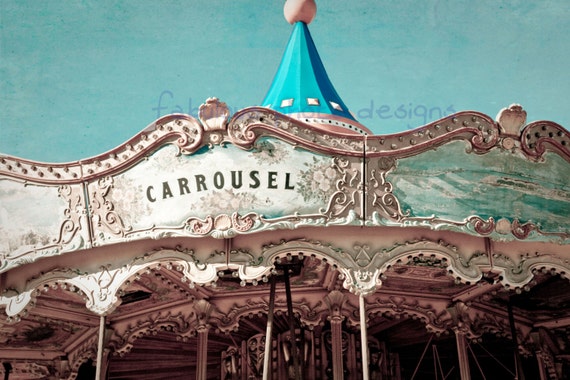The image depicts a nostalgically aged, vintage photograph focused on the top portion of a carousel. The colors in the photo are slightly faded, giving it a sepia-toned, old-timey feel. The scene captures intricate details of the carousel, showcasing its ornate design characterized by undulating swirls and bouquets of flowers around the word "carousel" written in black text. The dome top, resembling a birthday hat, is pyramid-shaped and colored blue with a pink sphere on top. This zoomed-in view encompasses the structure from the mid-poles, typically holding horses, upward. The sky in the background displays a rustic blue hue, enhancing the image’s nostalgic atmosphere.